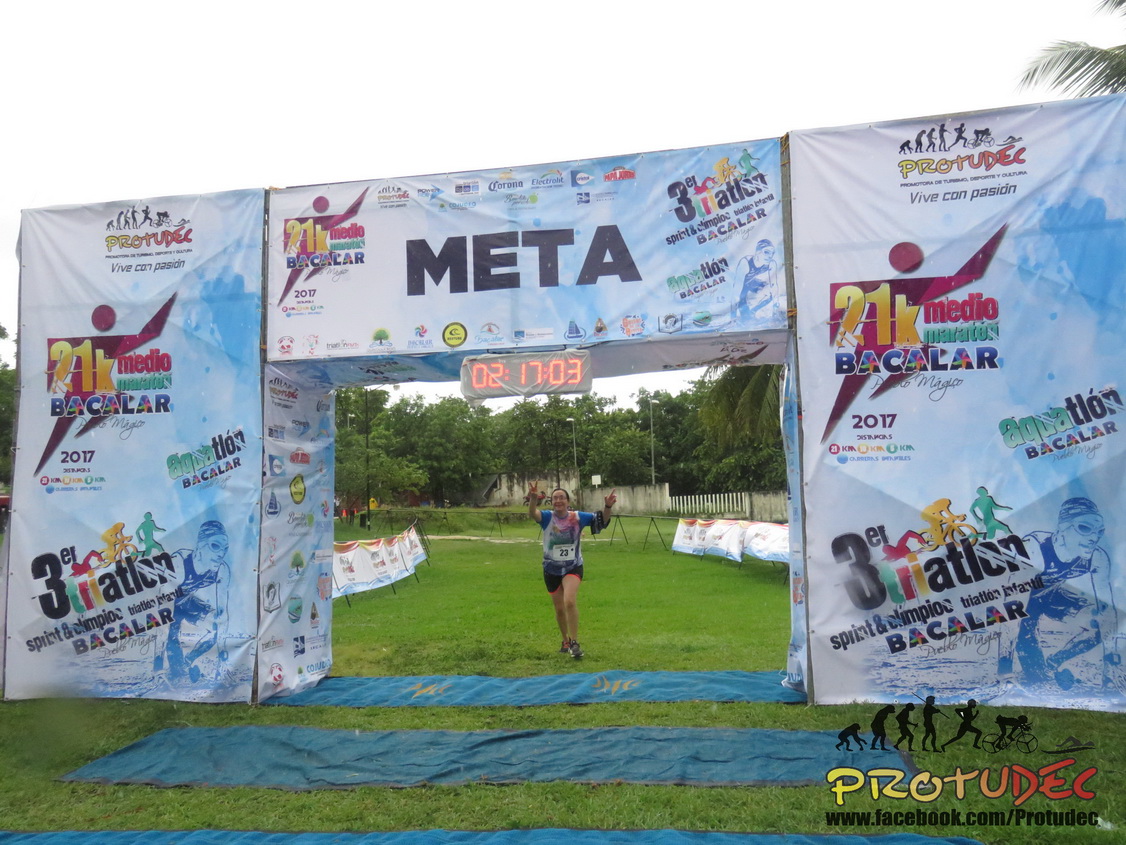The photograph depicts an outdoor marathon event on a gray, overcast day. The main focus is on the finish line arch, prominently displaying the word "META" in bold black letters, indicative of Spanish-speaking regions. Various colorful sponsor banners including "Aquathlon Baccalaureate," "3ER Triathlon," and "Sprint and Olympiak Baccalaureate" adorn the arch, creating a vibrant backdrop against the predominantly white and blue-colored arch banners. A digital clock hangs centrally from the arch, showcasing a time of 2 hours, 17 minutes, and 3 seconds in bright orange digits.

In the center of the image is racer number 23, a woman with light skin and her hair pulled back in a bun or ponytail. She is wearing a two-toned short-sleeved T-shirt with blue sleeves and a white front, along with black shorts. As she approaches the finish line, she joyfully raises both arms, forming a peace sign with her right hand while her left hand appears to be attempting the same gesture. The finish line area is a grassy field with various rugs laid down, and in the background, a few runners and some sparse trees are visible. 

Notably, the bottom right corner of the arch features artistic silhouettes depicting evolutionary progression—from a chimp to a standing man, then a running man, a cyclist, and finally a swimmer—emphasizing the multifaceted nature of the event. Below these silhouettes, the word "Protudec" is written in a gradient from yellow to red alongside its Facebook URL, adding a modern digital touch to the time-honored athletic event.